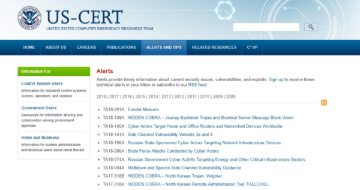This image depicts the homepage of the United States Computer Emergency Readiness Team (US-CERT) website. At the top, there is a partially visible green banner. Beneath it, a horizontal navy rectangle spans the width of the page, containing clickable links labeled "Home," "About Us," "Publications," "Reports," and "Resource Center." Below this, a larger green section is divided into three segments. In the center of the page, a prominent red "Alerts" label draws attention, indicating important updates. As you scroll down, the page features multiple blue hyperlinks, offering access to various resources and information. The background includes areas of white space, providing a clear and organized layout.